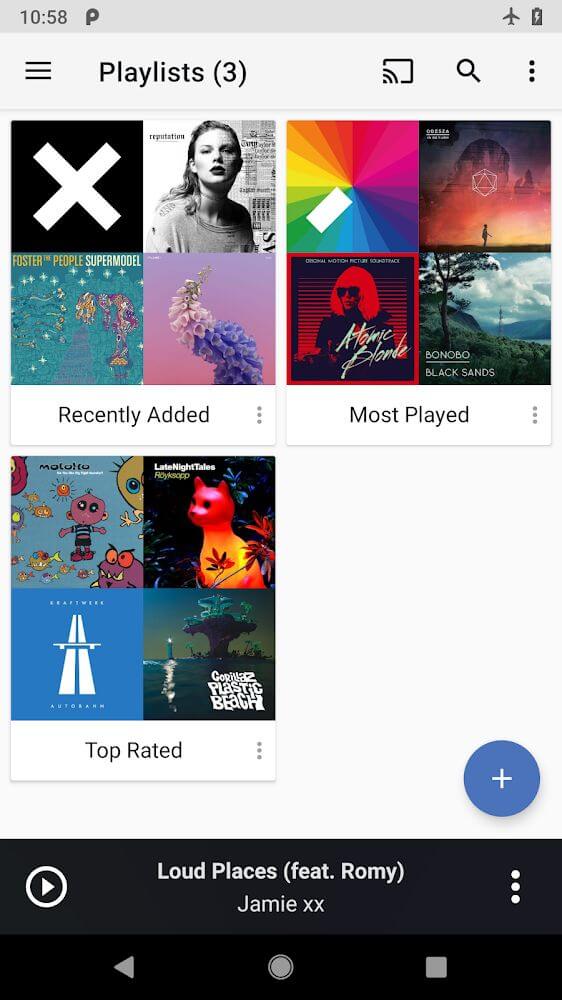This detailed screenshot from a mobile phone showcases the navigation and playlist interface of a music application. 

At the top of the screen, a dark gray status bar displays the time as 10:58, along with status icons indicating the phone is on airplane mode and is currently charging. Below the status bar, a navigation menu is represented by three horizontal lines on the left. To its right, the text "Playlists (3)" is prominently displayed, and further right are three icons: a Wi-Fi on tablet symbol, a search magnifying glass, and three vertical dots for more options.

The main portion of the screenshot is dominated by three playlists, organized in a 2x2 grid, leaving the bottom-right corner empty as white space. 

- The upper left playlist, titled "Recently Added," showcases four album covers: 
  1. The top cover features a white "X" on a black background.
  2. Below it is a photo or portrait of a woman.
  3. The third cover appears to be Foster the People's "Supermodel," recognizable by its vibrant and modern artwork.
  4. The last cover in this playlist displays an abstract, snake-like plant design.

- The upper right playlist, titled "Most Played," also contains four album covers:
  1. The first cover is a rainbow-colored geometric pattern.
  2. The second features a person standing before a sunset with a city in the background.
  3. The third is the "Atomic Blonde" soundtrack.
  4. The final cover is Bonobo's "Black Sands," depicting a serene forested island.

- The bottom left playlist, titled "Top Rated," displays five covers:
  1. A cartoonish Motoko album cover.
  2. The "Late Night Tales" compilation.
  3. "Floppy Cats," with a red and yellow illuminated cat illustration.
  4. An artwork resembling an airport runway with a bench in the foreground.
  5. "Gorillaz Presents Copillar Plastic Beach," depicting a blend of an island and an offshore drilling rig.

At the bottom of the screen, the currently playing song "Loud Places feat. Romy" by Jamie xx is shown in white text against a black background. A play icon is situated on the left, three vertical dots on the right, and the usual control buttons for the phone at the very bottom.

This comprehensive view allows an intricate look at the playlist organization and multi-faceted music library management on the mobile device.